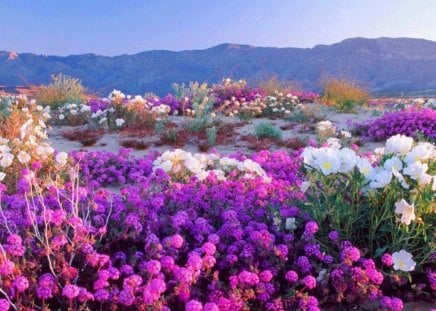The photograph showcases a vibrant outdoor flower garden set against a picturesque background. Dominating the bottom portion of the image, there is a lush array of bright pink and purple bell-shaped flowers. Among them on the right, white flowers with yellow centers rise on tall green stems. Moving towards the middle of the frame, a thin, sandy patch of light tan ground appears, interspersed with sparse greenery and small red accents. Behind this sandy area, a variety of flowers in pink, white, and purple hues form a colorful mosaic. The backdrop features a serene scene with gentle, grayish mountains that possess tinges of blue and purple, topped by a sky transitioning from a pale blue to a gradient of white. This sky occupies about the top fourth of the photograph, seamlessly framing the floral display. The mountains offer subtle details of green vegetation, adding to the landscape's depth and beauty.